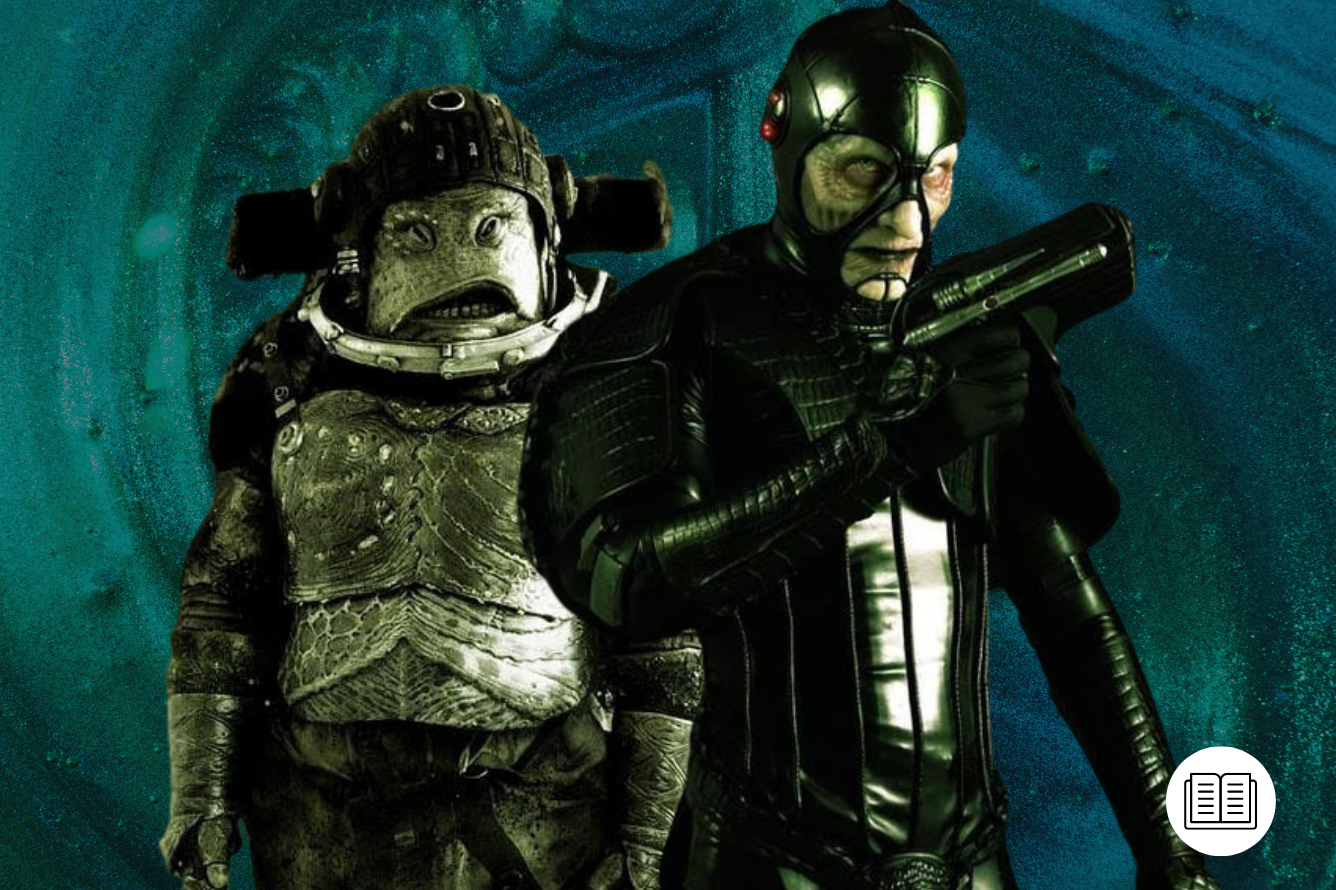In this highly detailed image, likely from a science fiction movie or video game, we see two distinct characters standing against a vivid, abstract blue wall that features a complex design. On the left side is an alien-like figure with a thick, fat appearance and a greenish skin tone. This character lacks a nose and has two eyes and a mouth visible. He is dressed in green and black clothing, accessorized with a matching helmet and armor, giving him a robust look. To his right stands a more human-like figure, though his face has a reptilian quality. He is fully clad in sleek black clothing and body armor. His helmet reveals only his eyes, nose, and mouth. In his right hand, he wields a futuristic black gun, possibly a laser weapon. This figure's attire and weapon contribute to his formidable presence. At the bottom right corner of the image, a black and white circular logo featuring a drawing of a book is present, hinting at some form of narrative or lore behind the scene.